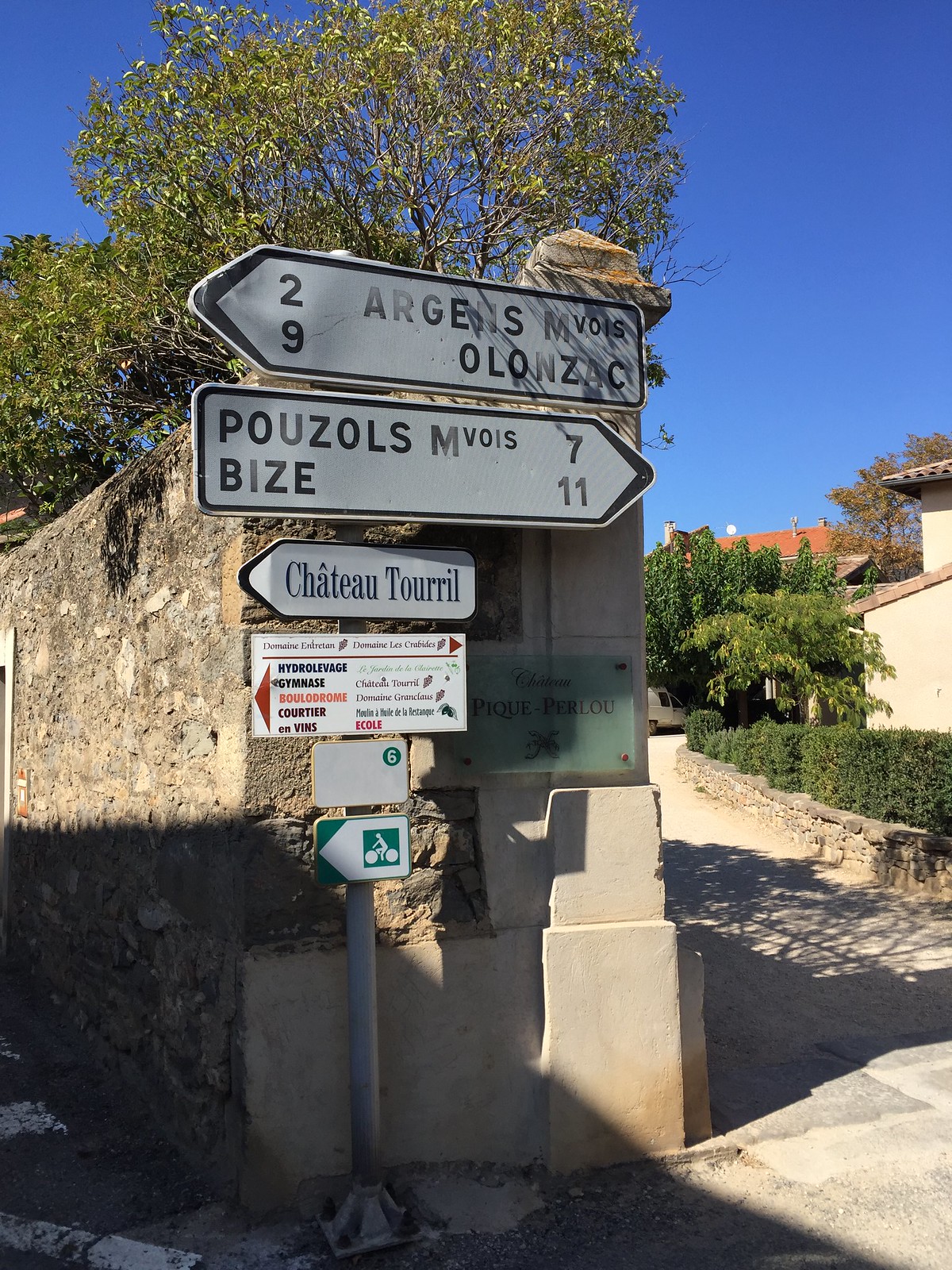This image depicts a picturesque road junction marked by a stone wall constructed of brownstone and a cement post adorned with multiple directional signs. Dominating the scene are two primary white signs with black borders and raised black lettering. The uppermost sign, pointing left, indicates "29 RGELS" with the letters "O-L-O-N-Z-A-C" underneath, suggesting a destination 29 kilometers away. Below it, a sign points right to "POUZOLS" and "BIZE," listing distances of 7 kilometers and 11 kilometers, respectively.

Beneath these main signs, a smaller sign directs left to "Chateau Teril." Below it, several other small, mostly illegible signs cluster on a metal pole extending from the ground, which appears to be cement. To the left and right of the central post, roads diverge, framed by lush trees and leading into the background where houses, including a little chateau on the right, subtly emerge from the scenery.

Additional intriguing details include a smaller white square sign with unreadable text and a distinct white sign featuring a red arrow on the left and possibly a green "6" or "S" mark. At the bottom of the array is another sign displaying an arrow and an icon of a person riding a bike. This diverse collection of signage elegantly orchestrates the navigation of travelers through this quaint, tree-lined crossroads.